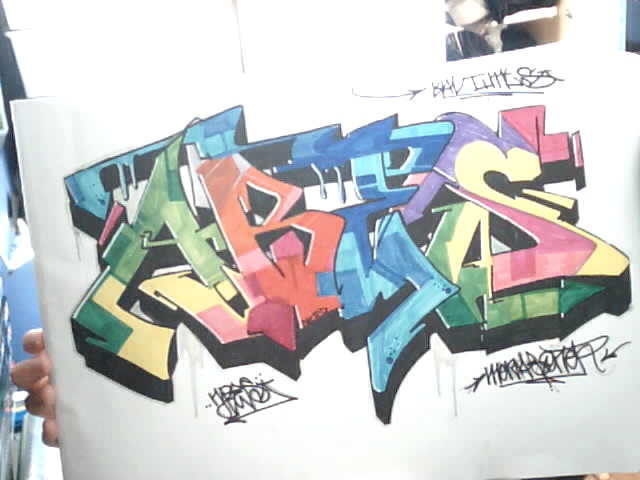This photograph captures a vibrant piece of urban artwork, likely graffiti, presented on a sheet of paper. A hand on the left side of the frame holds the paper, revealing slight wrinkles that suggest its material. The artwork features a dynamic blend of high-energy letters that are difficult to fully decipher but appear to include characters like A, B, R, T, and S. The colors used are striking and varied, including shades of green with yellow stripes, orange, yellow, pink, bright red, dark red, and multiple hues of blue ranging from powder blue to dark blue. The letters are designed in a three-dimensional style, accentuated with black shadows that add depth. Below the main artwork are two signatures of the artist, with an additional signature appearing above the letters. This graffiti-like creation exudes the fast-paced, kinetic energy typical of urban art often seen on city streets or railway cars.